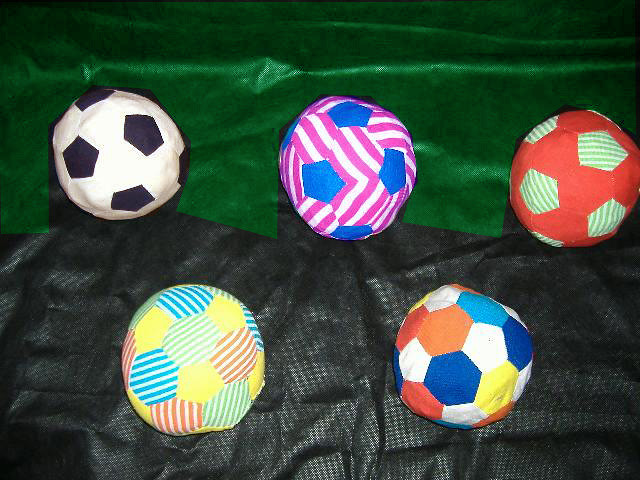This color photograph showcases a collection of five soft, pillow-like soccer ball toys arranged in a pattern reminiscent of the Olympic rings. They are placed in two rows on two different types of fabric. The top row features three balls equidistant from each other, lying on a dark green, shiny fabric that appears to be velvet. The bottom row has two balls situated on a black, textured, and crumpled material with a small perforated design. The soccer ball on the upper left is white with black pentagonal patches, resembling a traditional soccer ball. The ball in the middle of the upper row has white and pink stripes with blue patches. The ball on the upper right is orange with green and white striped patches. On the bottom row, the left ball features a variety of pastel patches with stripes in colors such as blue, white, green, pink, and white. The ball on the bottom right is adorned with multicolored patches—white, blue, orange, yellow, red, and a brighter blue.